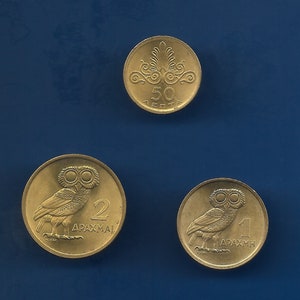The image features three distinct coins arranged in a triangular formation against a dark navy blue background. The top coin, slightly tarnished and about the size of a nickel, displays a filigree ornamentation, possibly floral, and is inscribed with "50 E-N-T" or "50 cents." Positioned below, the bottom left coin is larger, resembling the size of a quarter, and depicts an etched owl with the number "2" beside it, accompanied by the inscription "APAXMAI." The bottom right coin, slightly smaller than the left one and closer in size to a nickel, also showcases an owl with the number "1" next to it, bearing the same inscription, "APAXMAI." All coins appear to be crafted from a brass or gold-like metal.